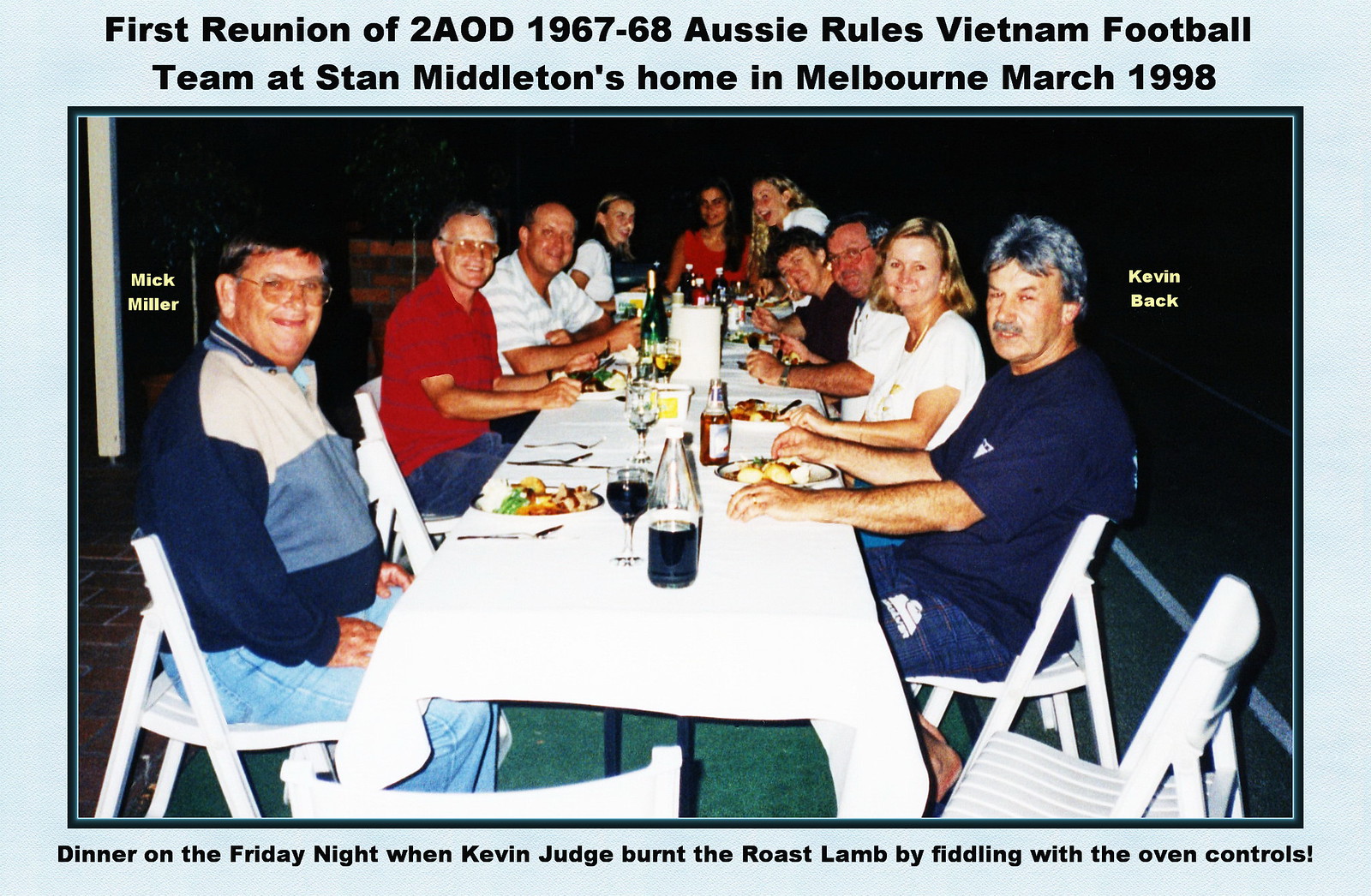This photograph captures a lively reunion of the 2AOD 1967-68 Aussie Rules Vietnam football team, held at Stan Middleton's home in Melbourne in March 1998. The image shows a long table adorned with food and drinks, where at least ten people are seated, smiling, and looking at the camera. The individuals are mostly sitting on either side of the table, with four people on the left side and four on the right, while two occupy the head of the table.

Names have been typed and placed at the head of the table for two attendees: Mick Miller on the left side and Kevin Beck on the right side front. Everyone in the photograph appears to be enjoying the occasion, with a sense of camaraderie visible in their expressions. The top label of the photo notes the significance of the event as the first reunion of the team, while the bottom label humorously recalls an incident from the evening, mentioning "dinner on Friday night when Kevin burnt the roast lamb by fiddling with the oven controls.” This detailed glimpse into their reunion highlights the warmth and shared memories of the group.